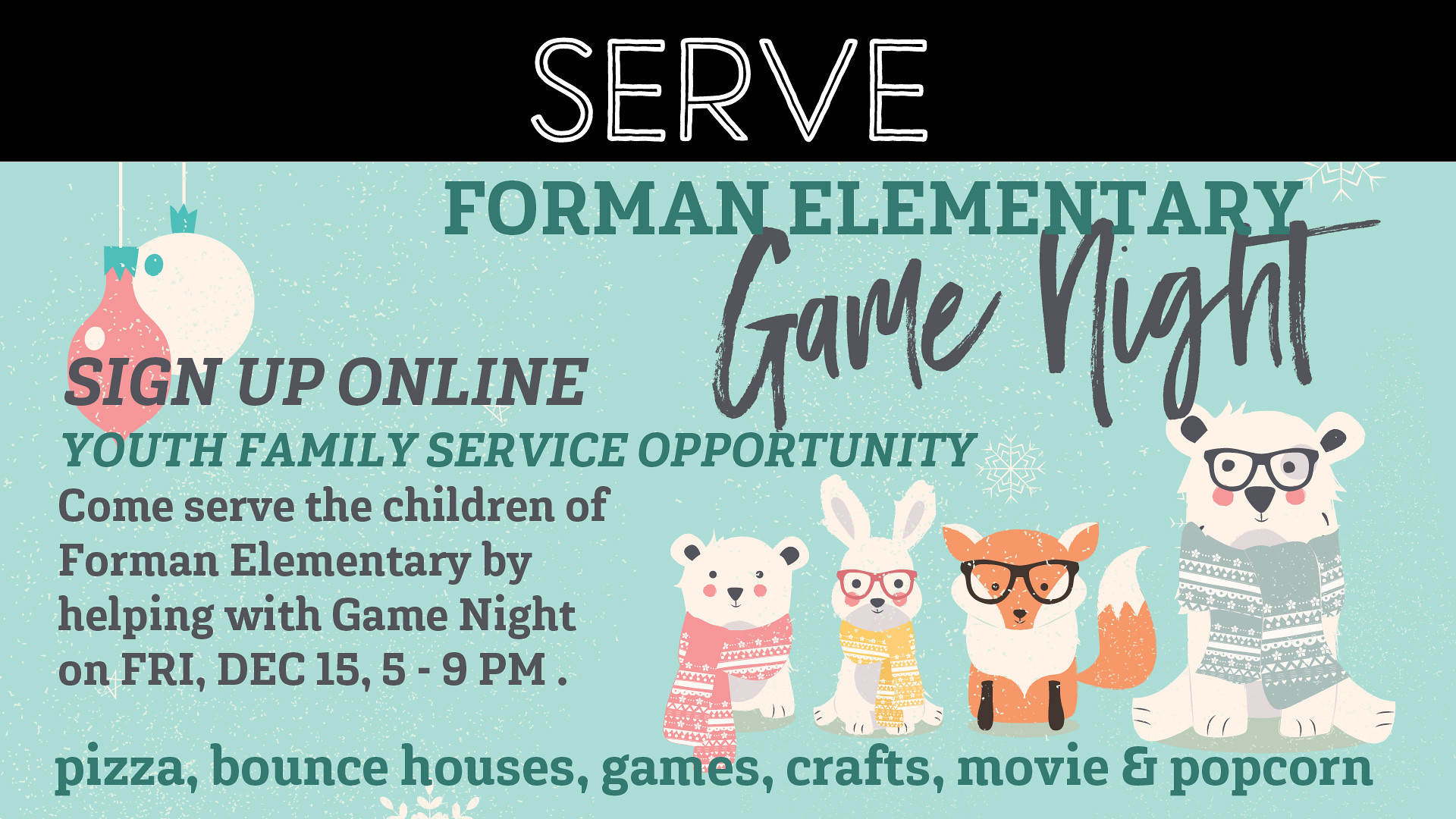This flyer advertises a game night event hosted by Foreman Elementary, prominently inviting families to sign up online. At the top of the poster, set against a black strip with white "SERVE" lettering, it reads "Foreman Elementary" in a darker green over a light green background that occupies most of the poster. Below, in an elegant black script, it states "Game Night" with further details including a youth family service opportunity, encouraging participants to help serve the children. The event is slated for Friday, December 15th, from 5 to 9 p.m., and promises an evening filled with pizza, bounce houses, games, crafts, a movie, and popcorn, highlighted in gold font. To the right, there are delightful illustrations of four cartoon animals – a bear, a bunny rabbit, a fox, and a dog – all wearing cozy sweaters, three of them donning glasses. The lower right corner features the animals, while the upper left showcases festive Christmas ornaments, reinforcing the holiday season theme.